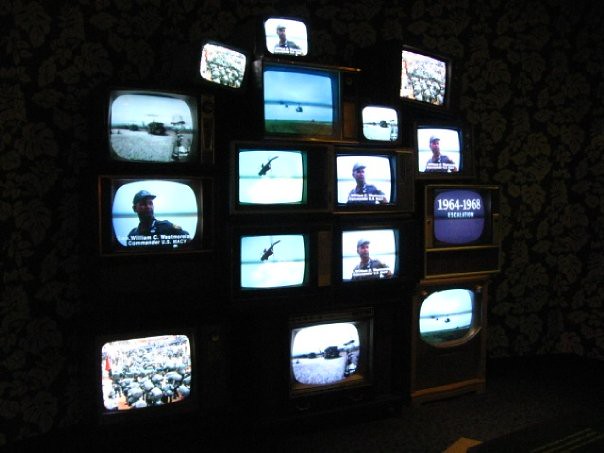This photograph showcases an array of 16 old-school television sets arranged in a nearly circular formation on a dark wall adorned with white flower designs. The predominant color in the image is black, accentuated by the glowing screens. The TVs vary in shape, with some having rounded edges and others featuring square screens. These screens display a range of images with varying degrees of color saturation. Notably, multiple screens depict a man wearing a black cap accompanied by captions beneath him. Other screens show diverse images such as birds, stones or rocks, and a sea scene. One particularly notable screen on the right indicates years "1964 to 1968" beside an image of a flying object. The scene is strikingly illuminated only by the television screens, casting a unique light in an otherwise dark room. The nostalgic design of the TV housing evokes memories of childhood for many viewers.